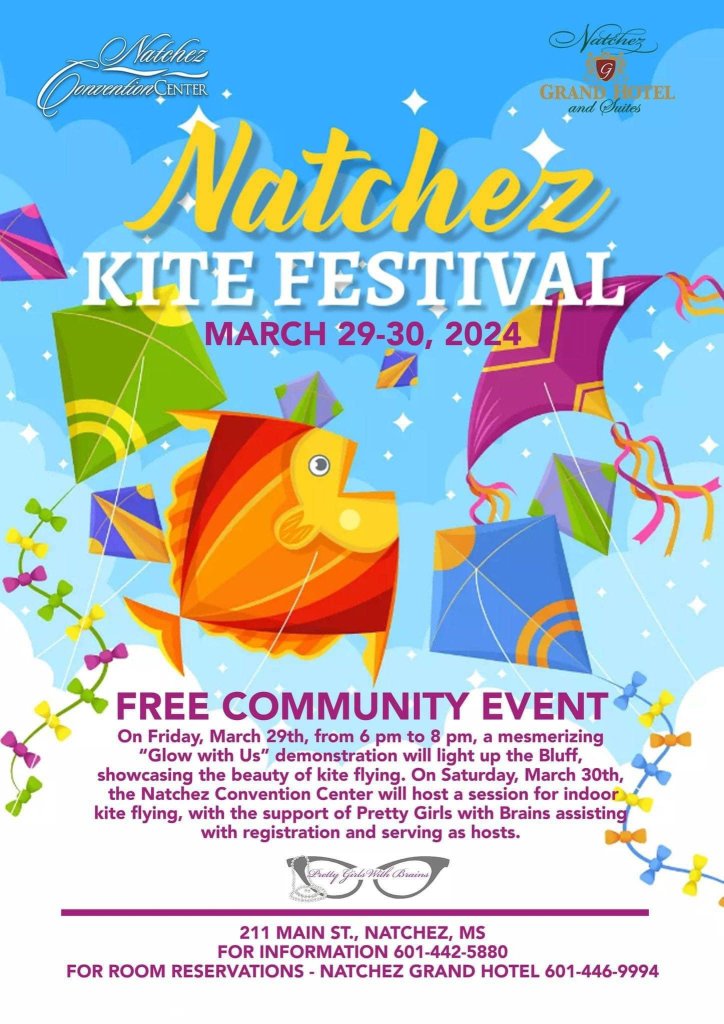The poster advertising the Natchez Kite Festival is a vibrant and colorful display set against a mostly blue sky with varying shades of blue to represent clouds. The event is scheduled for March 29-30, 2024 and is a free community event. Located at 2111 Main Street, Natchez, Mississippi, the poster provides a phone number for further inquiries as well as reservation details for staying at the Natchez Grand Hotel and Suites. Prominently featured at the top are the names "Natchez Convention Center" and "Natchez Grand Hotel and Suites." The kites depicted in the background are of multiple shapes and sizes, showcasing bright, rainbow-like colors including green, orange, red, blue, and purple. A prominent kite shaped like a giant goldfish is illustrated in the foreground, while other smaller kites with diverse designs such as two half circles and colorful paper tails appear scattered across the sky. The flyer further includes additional details about the festival within a descriptive paragraph.